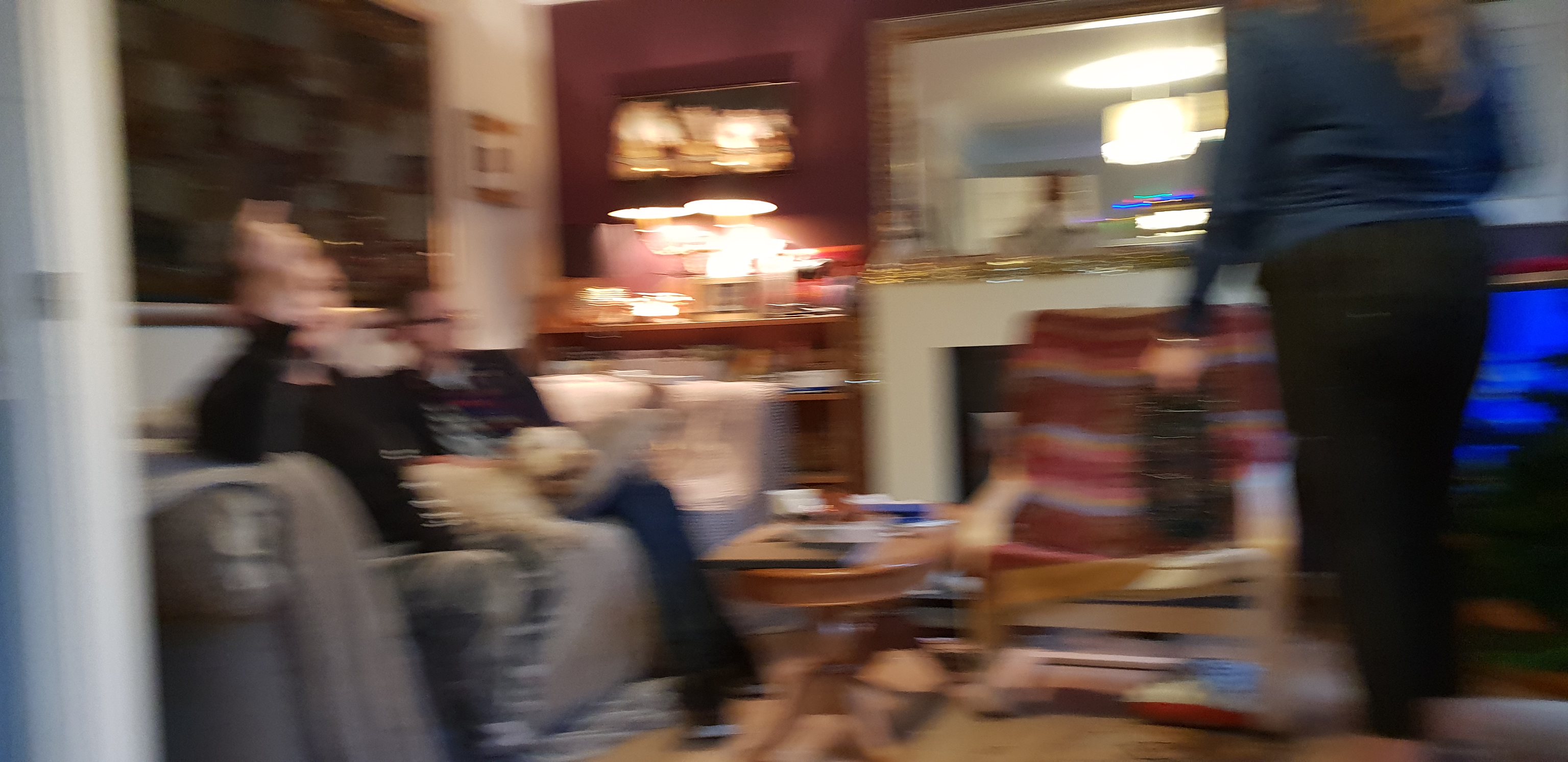In this extremely blurry photo of a cluttered living room, the scene is filled with numerous indistinct yet identifiable elements. On the left side, a gray or possibly white leather couch seats two people, one of whom is wearing blue jeans and appears to have a golden dog resting on their lap. Behind them, there is a large black-framed painting or a pattern on a black curtain, it’s too unclear to ascertain. To the right, a woman with mid-back length reddish-blonde hair, clad in a dark blue long-sleeve shirt and black pants, is standing. The room features a wooden chair in the center adorned with a striped blanket of red and blue hues. Nearby, there appears to be a very small, cluttered coffee table and a wrinkled rug on the floor. The back wall holds either a mirror with a gold frame, a fireplace, or a paneled area filled with lights and knickknacks, accenting the chaotic yet homely atmosphere.